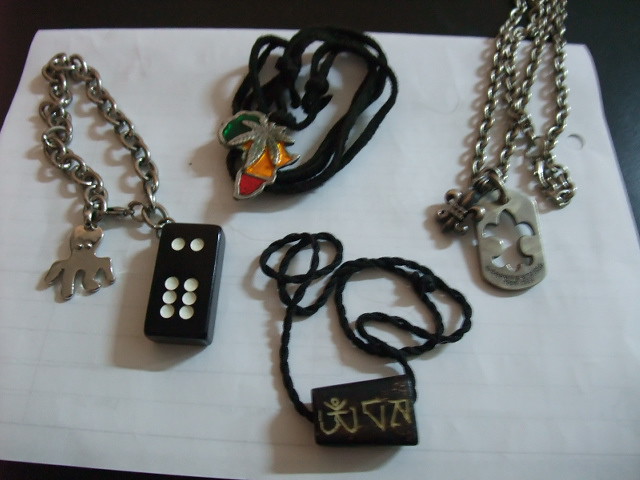The image showcases a collection of jewelry pieces arranged on a white piece of paper placed on a dark gray background. On the left side, there is a silver bracelet adorned with two charms: a detailed silver octopus and a black domino block featuring two white dots on the top half and six white dots on the bottom half. To the top right, there is a necklace made of black cord, intricately tied, supporting a pendant shaped like the continent of Africa colored in green, yellow, and red stripes with a silver marijuana leaf at the center. Adjacent to it, a heavy silver chain necklace displays a pendant with an ornate design, featuring a cut-out pattern resembling three elongated leaves with rounded ends. At the bottom, another black cord necklace holds an oblong brown pendant with white carvings that appear to include random letters or symbols, one of which resembles a head with arms raised.